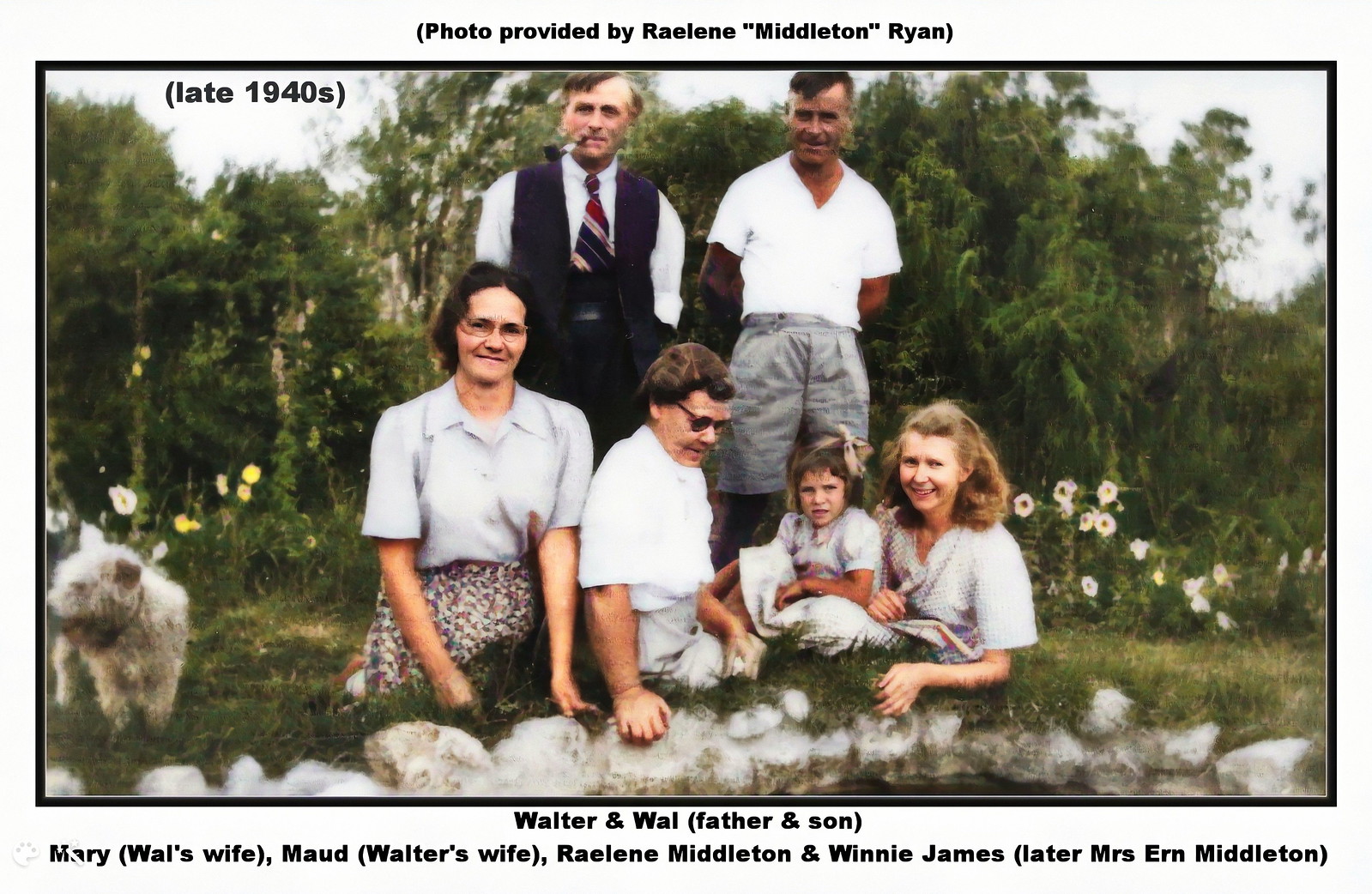This vintage family photo from the late 1940s, provided by Raylene Middleton Ryan, captures an intimate outdoor scene framed with a thin black border on a white background. The top left corner inscribes "late 1940s," aligning with the nostalgic essence of the black-and-white photograph. Below the image, detailed captions identify the family members: “Walter and Wall, father and son; Mary, Wall's wife; Maude, Walter's wife; Raylene Middleton; and Winnie James, later Mrs. Erin Middleton."

In the image, two men are standing side by side, each distinct in their attire. The man on the left, presumably Walter, sports a white button-down shirt with a red, blue, and white tie, complemented by a navy blue or black vest and matching suit pants. He also has a pipe in his mouth and short gray hair. Next to him, Wall wears a short-sleeved button-down white shirt paired with gray shorts.

Seated on the grass in front of the men are four women and a young girl. The far-left woman, possibly Maude, wears eyeglasses, a white short-sleeved button-down shirt, and a floral skirt. Beside her, Mary is visible in dark sunglasses and attired in a white button-down shirt with a gray skirt. The young girl, sitting on the lap of another woman potentially identified as Raylene, wears a long gray dress. Raylene herself sports a plaid short-sleeve top. A white, hairy dog is seen on the far-left side of the image, adding a touch of charm.

The backdrop brims with lush greenery, comprising tall bushes, trees with vibrant foliage, and a scattering of yellow and white flowers. This serene setting appears to be the family's backyard, with white rocks adorning a small pond nestled among the vegetation.